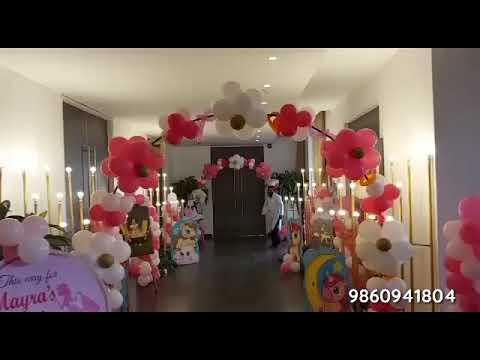The image depicts a banquet room intricately decorated for a celebration, possibly an event in honor of someone named Mayra, as indicated by partial text on the left side of the image stating "Myra's" with white balloons above it. Dominating the foreground is a large archway draped with balloon arrangements shaped to resemble flowers, primarily in pink and white, with some details suggesting accents of gold. Amongst these decorations, there are numerous bunches of balloons spread across the room. Deeper into the background stands a person clad in a white coat, possibly signaling a chef due to the white hat, or some sort of formal attire, positioned next to a three-candled candelabra which appears to have light bulbs at the top instead of actual flames. Behind this individual is a door or possibly an elevator door, contributing to the banquet room's ambiance. Additionally, near the person is a stand adorned with what looks like cartoon character stand-ups or props. Lower right of the image features a long number, 9860941804, adding a puzzling element to the scene.